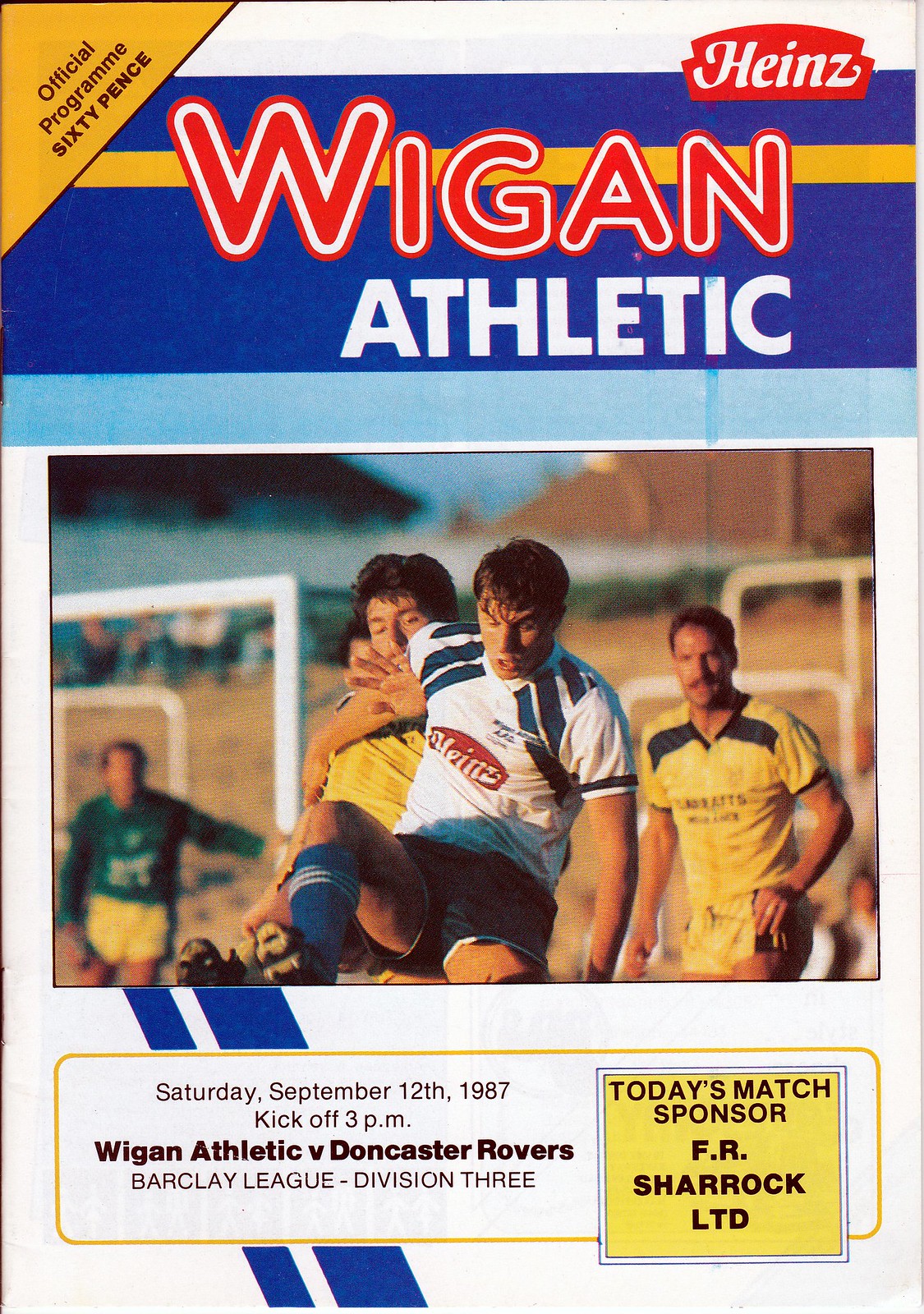This image is the cover of an official Wigan Athletic soccer match program priced at 60 pence. At the top right corner is a red Heinz logo with white letters. In the top left corner, there is a yellow triangle with "official program 60 pence" written in black text. Dominating the middle section, the title "Wigan Athletic" is prominently displayed, with "Wigan" in large red bubble letters and "Athletic" in white block letters. This title sits on a royal blue rectangle that has a yellow stripe running through the top third.

Below the title is a thinner, light blue horizontal bar, followed by a photograph of a soccer match. The photograph showcases four players: a guy in a white jersey with blue stripes and a Heinz logo, wearing black shorts; two players in yellow and black jerseys; and in the background, another player, a goalkeeper, stands at the left wearing a long-sleeve green shirt and yellow shorts in front of a white goal. 

At the bottom of the image, a white horizontal box contains black text detailing the event: "Saturday, September 12th, 1987, kickoff 3 p.m., Wigan Athletic versus Doncaster Rovers, Barclay League Division III." To the right of this, there is a yellow rectangle with black text that reads "today's match sponsor, FR Sherrock Limited." This detailed and colorful cover encapsulates the excitement and particulars of the Wigan Athletic versus Doncaster Rovers soccer match.